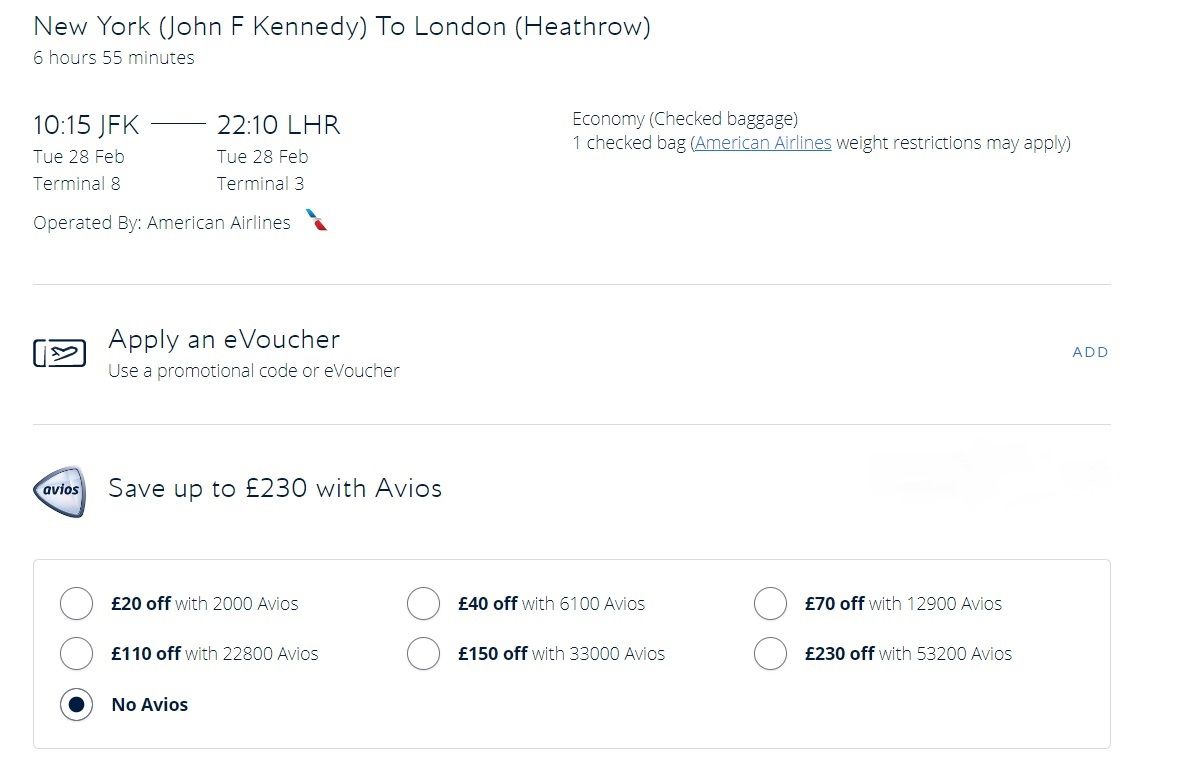Here is the cleaned-up and detailed caption for the image:

---

This screenshot displays a travel booking page focused on purchasing airfare. The main section at the top-left of the screen showcases details for a flight route from New York (John F. Kennedy International Airport, JFK) to London (Heathrow Airport, LHR). A blue dot indicator provides the flight duration, "6 hours 55 minutes," and highlights the departure and arrival times: 10:15 AM (JFK) to 10:10 PM (LHR). Directly underneath, the departure date is marked as Tuesday, February 28th. The respective terminals are mentioned next: Terminal 8 for JFK and Terminal 3 for LHR, with American Airlines operating this flight.

Additionally, the American Airlines logo is featured prominently below these details. There is an option to "apply an e-voucher." To the left of this option is a rectangular icon depicting an airplane, while to the right is the word "add," separated by a dividing line. Further down, there is a note indicating that travelers can "save up to 230 pounds with e-vouchers."

---